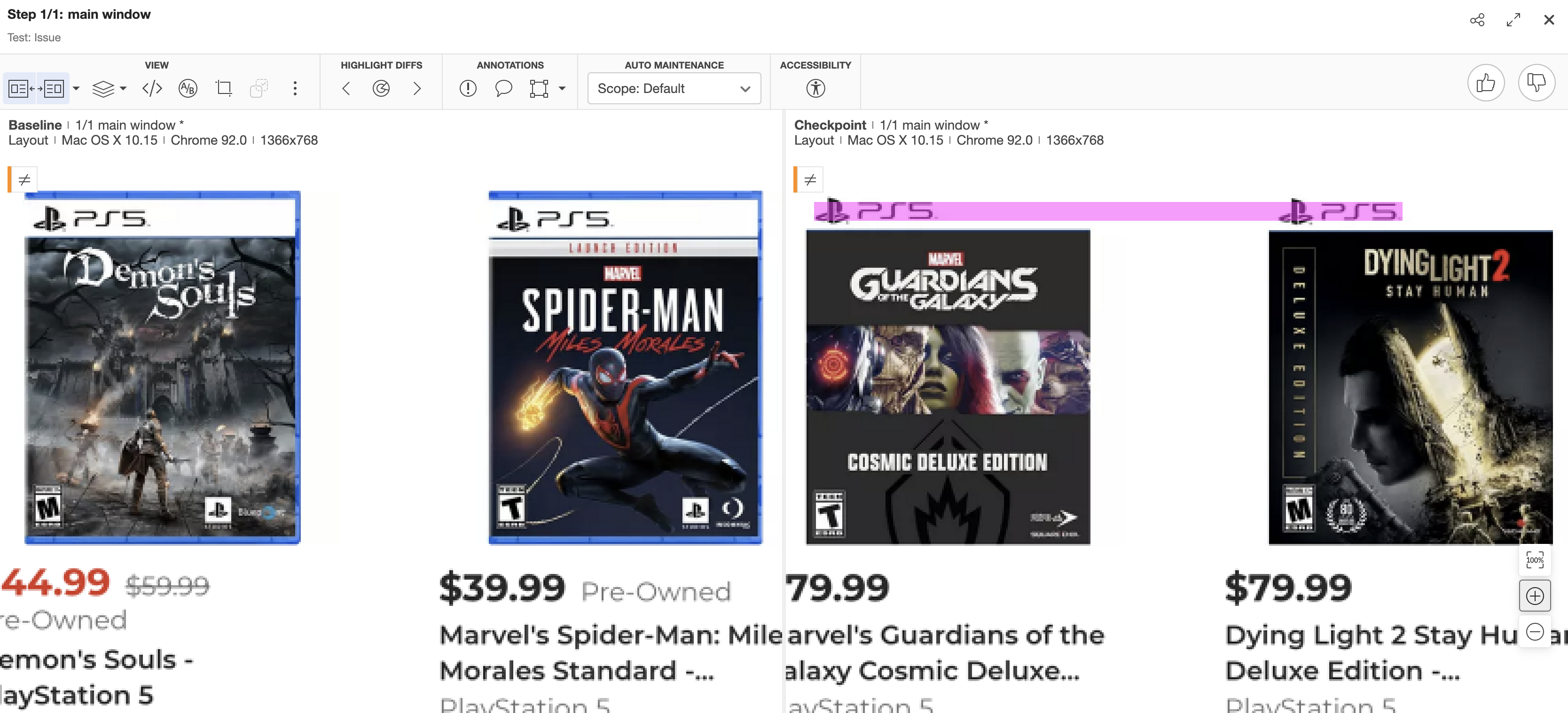This image is a screenshot of a website with a predominantly white background. At the top, it features the heading "Step 1/1: Main Window" with the 'S' in 'Step' capitalized. Adjacent to the heading are several icons, including three circles connected with lines, an arrow that ascends and descends diagonally, and an 'X'.

Beneath this heading is a gray banner displaying several options: "View," "Highlight Diffs," "Annotations," "Auto Maintenance," and a dropdown menu labeled "Scope," currently set to "Default." This section also includes "Accessibility" and, at the far right, two circles with thumbs-up and thumbs-down icons.

Lower down, the text "Baseline: 1 of 1, Main Window" is visible, followed by the system specifications "Layout: macOS, 10.15, Chrome 92.0." Further information includes "Checkpoint: Layout."

Further down, the content shifts to a list of games with their respective details and prices. The first game listed is "PS5 Demon's Souls," followed by "Spider-Man for PS5," "Guardians of the Galaxy: Cosmic Deluxe Edition" also for PS5, and "Dying Light 2: Stay Human" for PS5, with their prices displayed beneath each title.